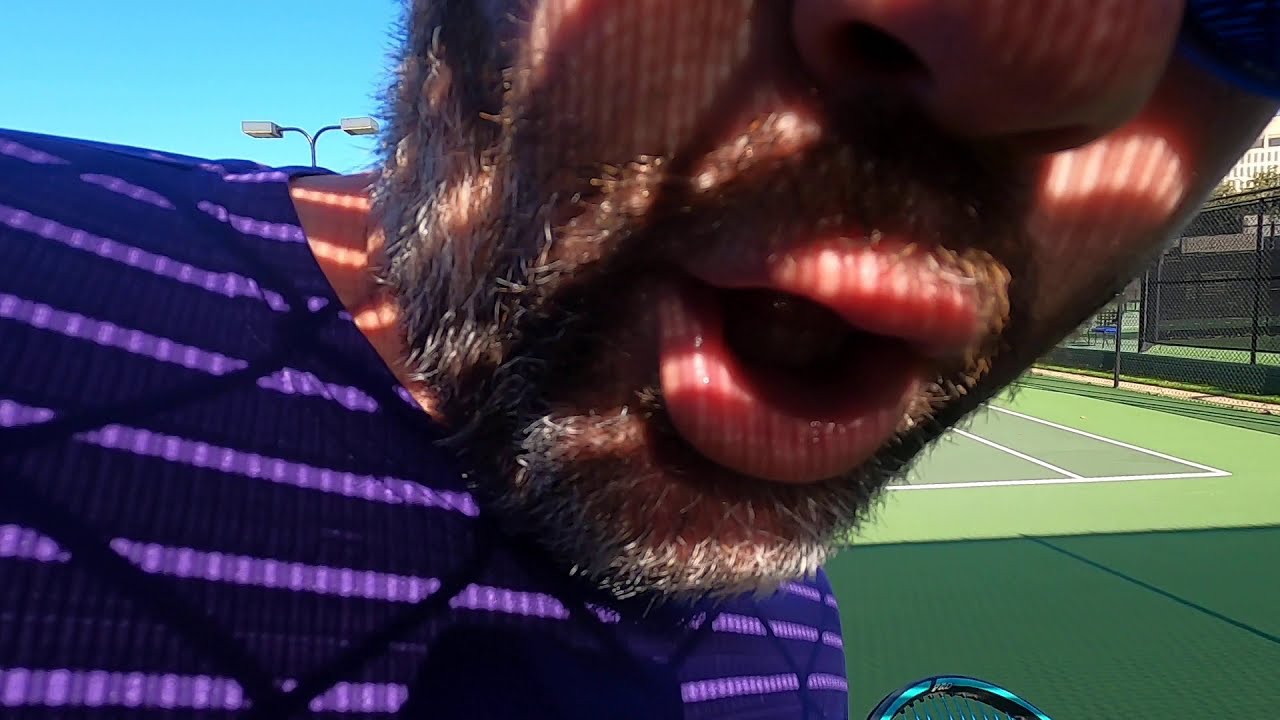The photograph is a striking, wide rectangular close-up focusing on the bottom half of a man's face, particularly his mouth, beard, and the lower part of his nose. His beard is salt-and-pepper, adding depth to his skin tones. He is tilting upwards and to the right, with his mouth slightly open. His torso, partially in view on the left side of the image, is clad in a distinctive purple striped shirt that catches the light, creating horizontal reflections. Shadows of a chain-link fence trace across his shirt, enhancing the outdoorsy atmosphere. 

In the background, a green tennis court bordered by a black fence occupies the lower left corner of the image, delineated with crisp white lines. Behind the court are a range of buildings suggesting urban surroundings. The upper right corner features clear blue sky and the top of a light post, indicating a sunny day. Additionally, in the lower right corner, the edge of an aqua blue and black tennis racket peeks into the frame, hinting at the activity engaging the man. The image successfully juxtaposes the detailed close-up of the man's face with the wider context of a serene, outdoor sporting area.